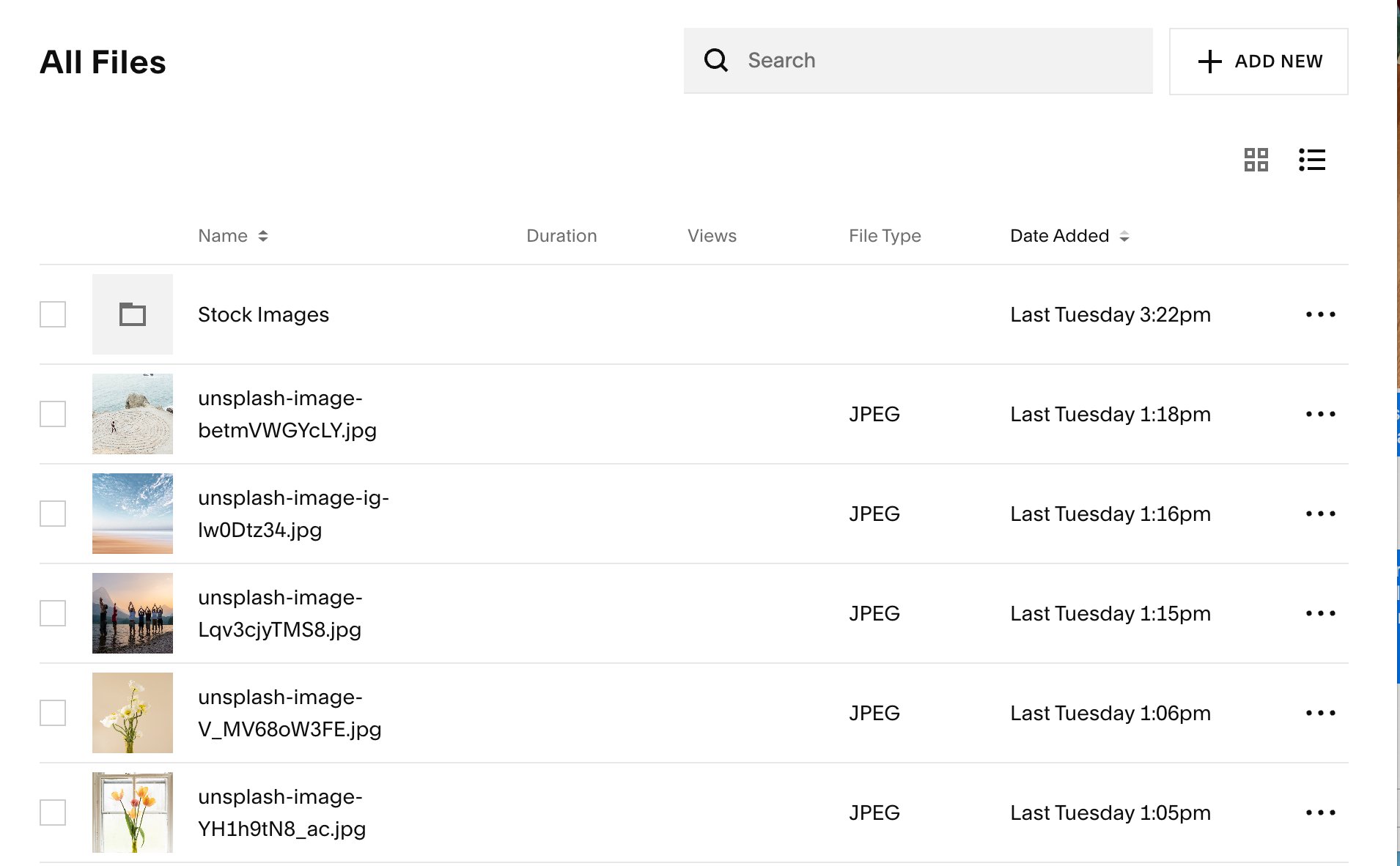In the image, we observe a file management program interface. At the top left corner of the screen, there is a header displayed in black text on a white background reading "All Files." Below this, the interface lists categorized columns labeled from left to right as: Name, Duration, Views, File Type, and Date Added. 

Proceeding further down, a horizontal row indicates a category titled "Stock Images," with a date added listed as "Last Tuesday, 3-22" but without additional details. 

Below this category, a sequence of small thumbnail images is visible. The first thumbnail, presumably of a beach scene, is labeled "Unsplash Image, JPEG, Last Tuesday, 1:18 p.m." The next thumbnail appears to be another beach scene, labeled "JPEG, Last Tuesday, 1:16 p.m." 

Following that, there is an image with several people raising their arms, which is also labeled "JPEG, Last Tuesday, 1:15 p.m." Further down, there are images that resemble flowers. The first flower image is labeled "JPEG, Last Tuesday, 1:06 p.m." and another flower image beneath it is labeled "JPEG Image, Last Tuesday, 1:05 p.m."